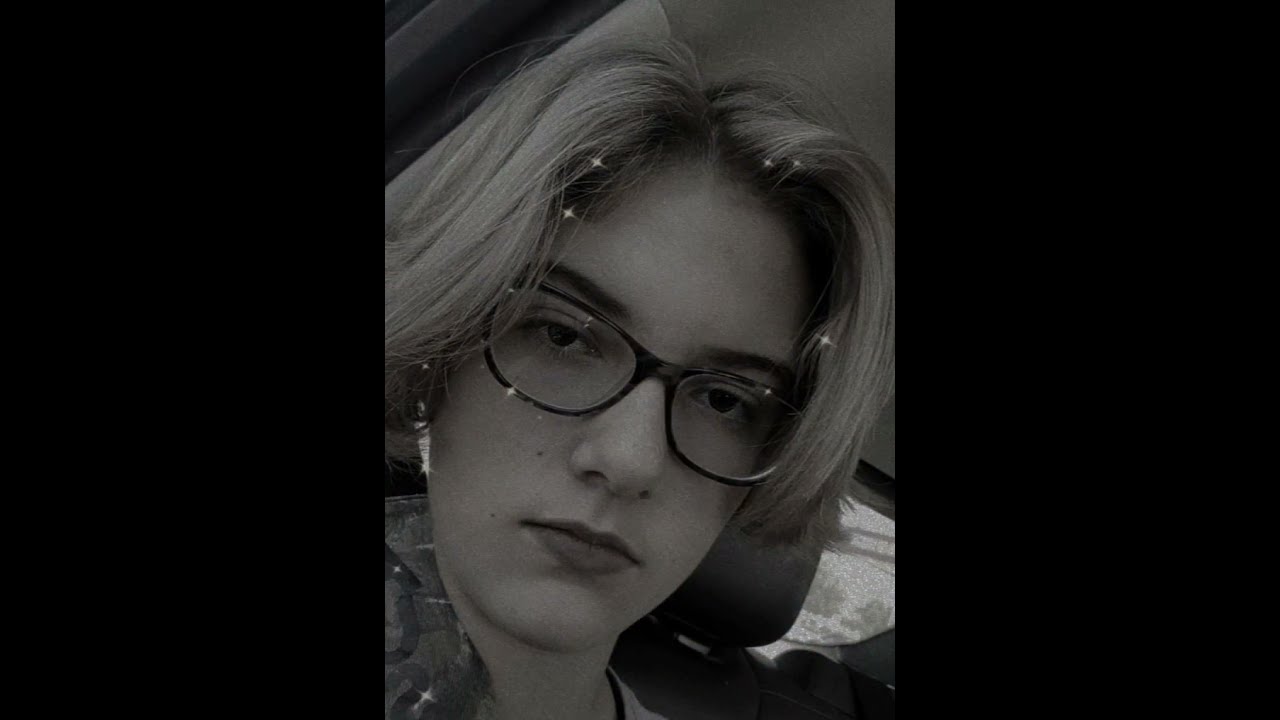The image comprises a three-panel design, with the left and right panels filled in solid black. Centered is a black and white photograph of a young woman with short blonde hair, styled around her face. She is facing the viewer directly with a stern, tired expression. Her dark-rimmed glasses frame her dark eyes, emphasized by her dark eyebrows and somewhat bulbous nose. The contrast between her thinner upper lip and fuller lower lip highlights her mouth, which shows no particular expression. She possesses a soft, rounded chin and wears what looks to be a shirt, possibly layered with a jacket. Silver earrings glint in her ears. Scattered across her face, hair, and glasses are digitally added white stars, giving the image a whimsical touch. In the background, the context of a car is implied by the visible back seat and rear window, suggesting she is seated inside a vehicle. The overall composition lends an introspective and slightly digital-enhanced feel to the photograph.